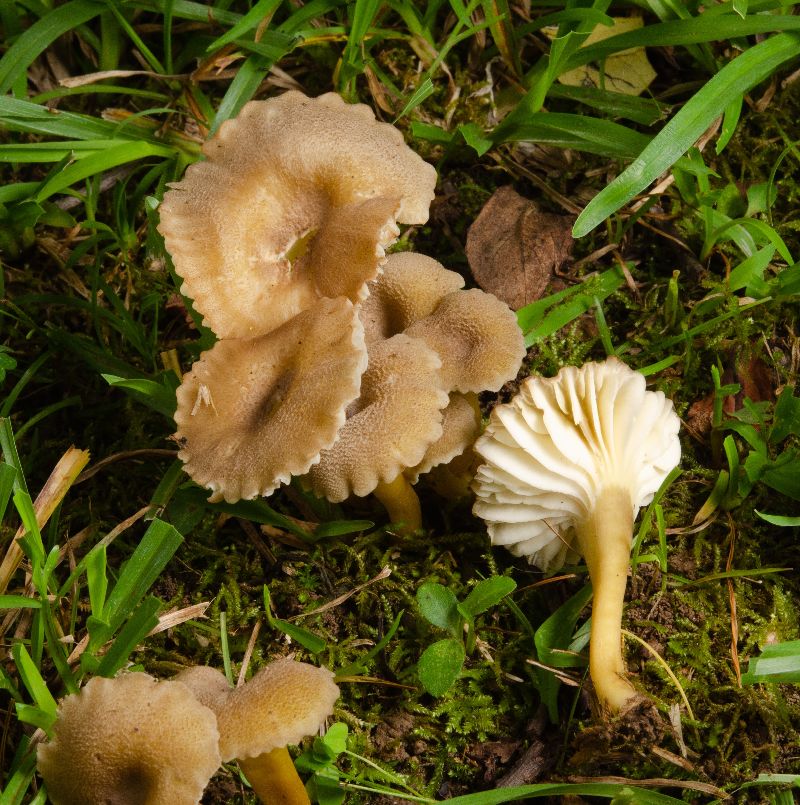The image is an extreme close-up of the ground, capturing a square foot area covered with dirt, grass, and brown leaves, indicating a natural outdoor setting. Prominently featured are around eight beige mushrooms, with brown caps and cream-colored gills underneath. These mushrooms are sprouting from various points in the ground. A noticeable cluster of four to five mushrooms is situated in the center, accompanied by a single mushroom lying on its side to the right, revealing its underside. Additionally, a small cluster of mushrooms can be seen in the lower left-hand corner, set against a backdrop of green grass and a few weeds, suggesting a summer scene.